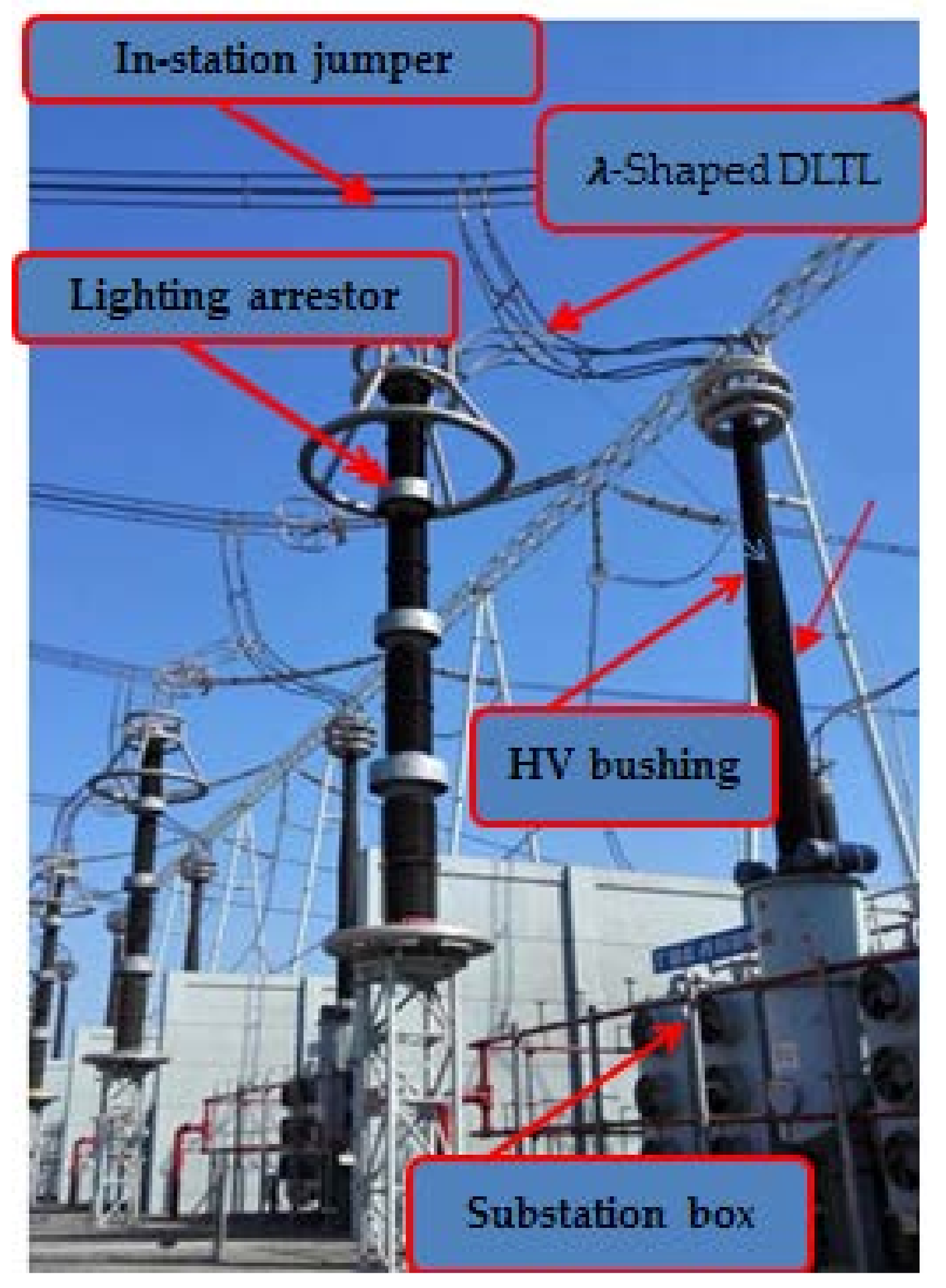This detailed color photograph depicts an electrical substation, a facility where power is stored and not generated. The image prominently features various electrical components and infrastructure, all amidst a clear blue sky. Numerous power lines stretch across the frame, connecting black poles and A-shaped towers surrounded by silver rings. The photograph is annotated with red text boxes containing blue interiors and black text, each accompanied by red arrows pointing to specific structures. These annotations label various parts of the substation: "In-station Jumper," pointing to the lines; "A-shaped DLTL," indicating the lines leading into a pole; "Lightning Arrester," aimed at a metallic circle around the poles; "HV Bushing," although somewhat unclear due to image quality; and "Substation Box," shown as a large area at the base of a pole with multiple nozzles. Additionally, a street sign is visible atop a chain-link fence bordering the substation. The overall machinery is predominantly silver and black, accented by black running wires and set against grayed-out walls, providing a comprehensive view of the substation's intricate electrical environment.